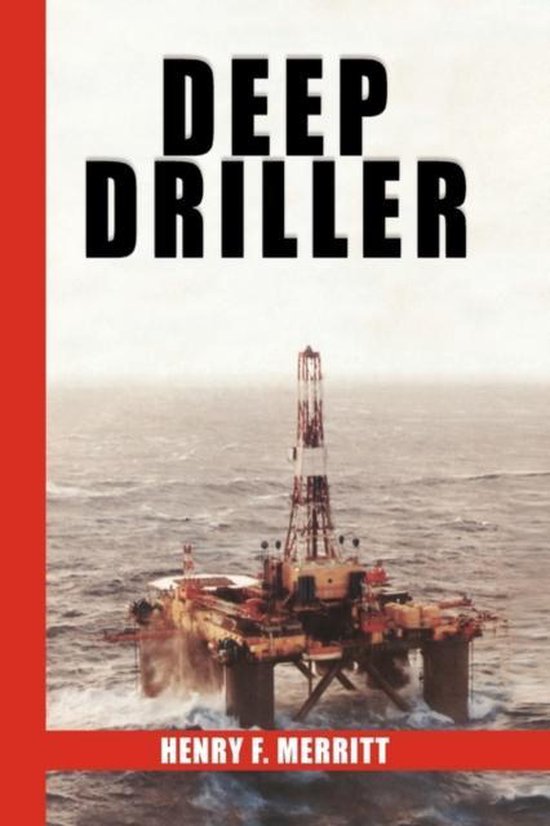This image appears to be the cover of a book titled "Deep Driller," set against an off-white, overcast sky. A bold red stripe runs vertically down the left-hand side and horizontally across the bottom, about a centimeter above the bottom edge. The author's name, Henry F. Merritt, is prominently displayed in capital white letters on the bottom red stripe. "Deep Driller" is written in bold black capital letters at the top, spanning from about 5% to 30% down the cover. 

The main visual feature is a color photograph of an oil rig situated in the middle of a vast, gray ocean with small waves splashing up around it. The ocean appears almost infinite, blending into the distant horizon. The rig itself, which resembles a miniature Eiffel Tower, stands on several large, rust-colored posts with remnants of white paint. It is constructed from metal, not wood, and shows signs of wear and rust, giving it a blend of red and brown hues. The sky above is a muted off-white, contributing to the overall desolate and industrial atmosphere of the scene.